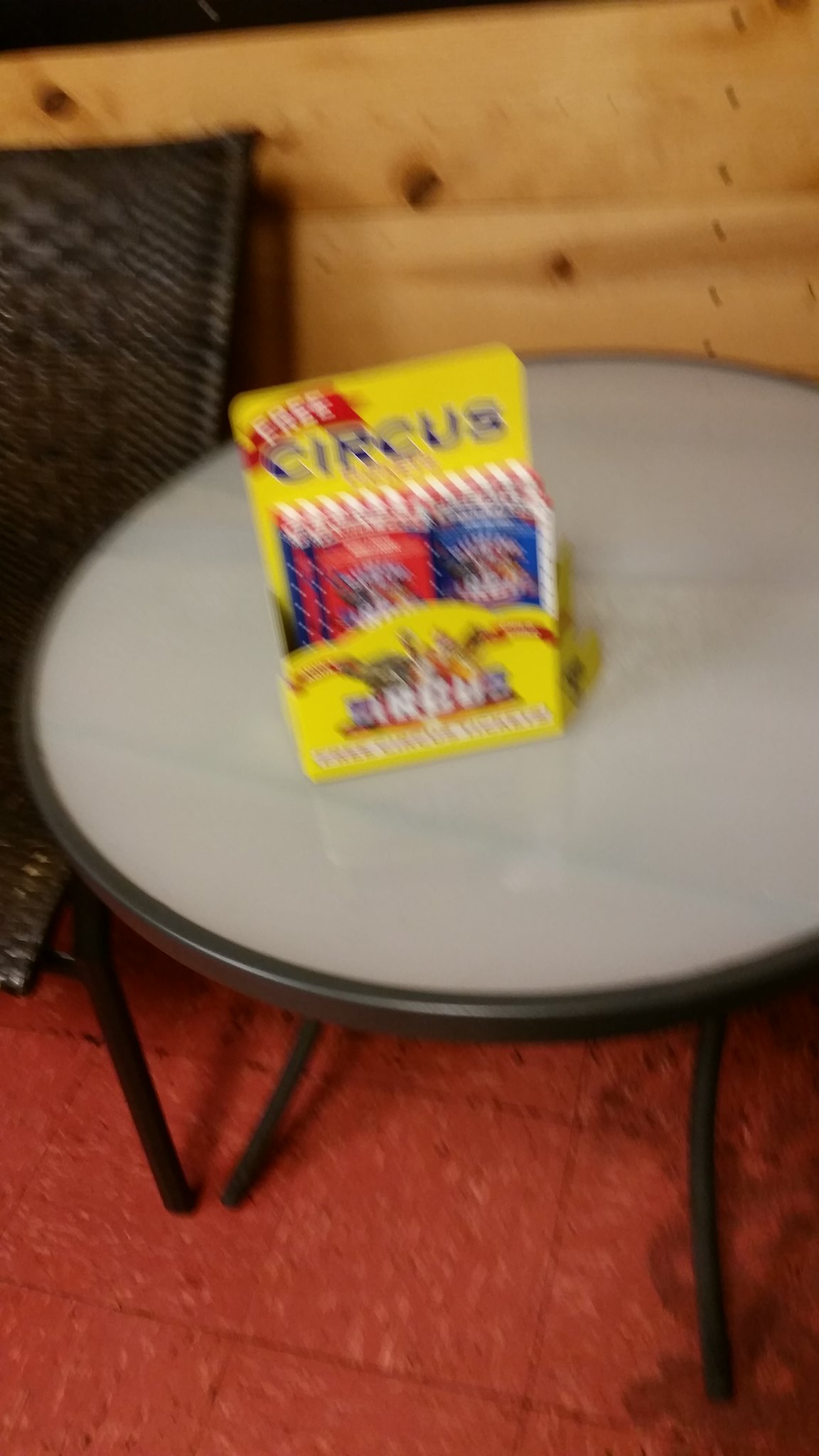The image depicts a somewhat blurry scene featuring a small, round bistro-sized coffee table placed against a lightly stained, honey-colored wood-grained wall. The table, characterized by its glossy and shiny light gray, pale white Formica surface, is supported by a black metal frame. Atop the table sits a conspicuous yellow box, adorned with the word "Circus" in blue lettering and a red banner above it declaring "Free". Although the image's blur obscures specific details, the box appears to contain several small booklets or packs of cards. Below the table, the floor is covered in red tiles with white flecks. To the left side of the image, a piece of dark furniture is partially visible, resembling a black basket-weave hardback chair.